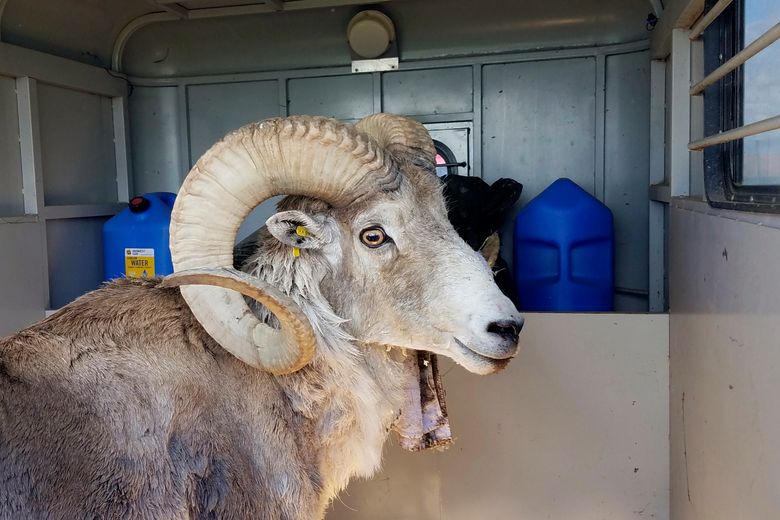The photograph depicts a ram standing in a silver, metal trailer or holding cell, characterized by a window with bars on the right side. Behind the ram, there are several blue containers, possibly gas canisters, and an indistinct black object. The ram has a predominantly white face with a light brown body, transitioning to a whiter underbelly. Its most striking feature is its large, curled horns, which form an S-shaped loop extending backward. The ram is facing slightly towards the right and has a yellow tag in its ear. It seems to be in a well-maintained, possibly man-made habitat, and while its expression is neutral, it exudes a sense of calmness.